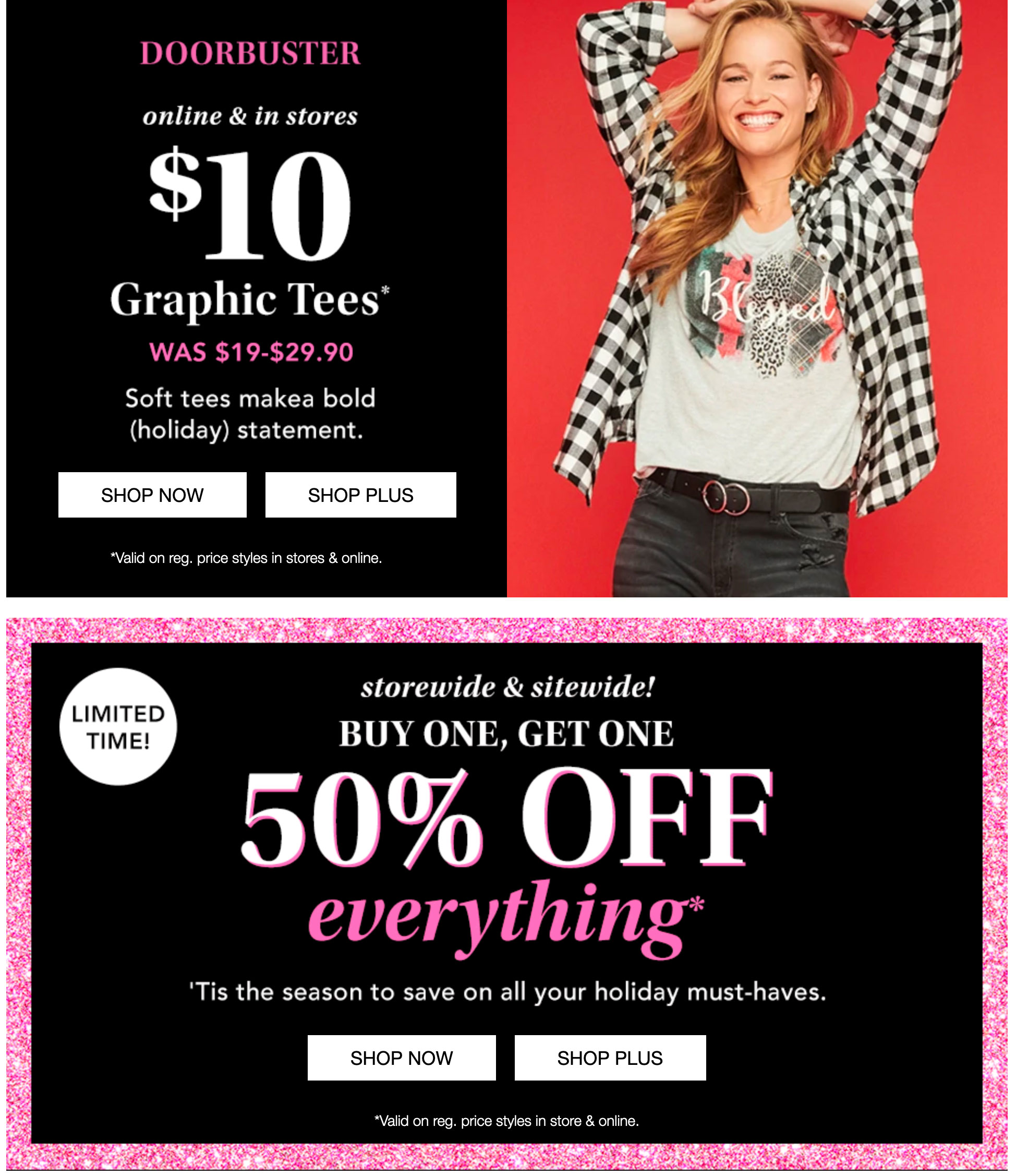The image features two overlapping graphics vertically aligned. 

**Top Graphic:**
- **Left Section:**
  - **Background:** Black
  - **Text:**
    - "DOORBUSTER" in rosy pink, uppercase letters.
    - Underneath, in white: "Online and In-Stores"
    - "$10" followed by "graphic tees" (was $19 to $29.90)
    - "Soft Tees Make a Bolt (Holiday) Statement" in white.
  - **Buttons:** Two clickable banners - "Shop Now" and "Shop Plus"
  - **Footnote:** An asterisk leading to "Valid on regular price, styles, in-stores, and online."
- **Right Section:** 
  - **Background:** Red
  - **Image:** A girl from the waist up, wearing a t-shirt, an open button-down long-sleeve shirt, and jeans.

**Bottom Graphic:**
- **Background:** Black with a pink border
- **Top-Left Circle:** "Limited Time"
- **Text:**
  - Center: "Store-wide and Site-wide. Buy one, get one, 50% off everything."
  - Additional Text: "Tis the season to save on all your holiday must-haves."
  - **Buttons:** "Shop Now" and "Shop Plus"
  - **Footnote:** "Valid on regular price, styles, in-store, and online."

This comprehensive image promotes a holiday season sales event, highlighting discounted graphic tees and a buy-one-get-one offer with emphasis on timely shopping both online and in-store.